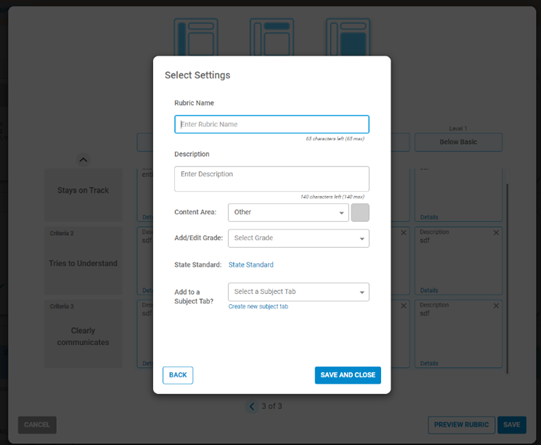The image features a detailed user interface for creating and editing a rubric. In the foreground, several input fields and options are prominently displayed. Users can specify settings, assign a name to the rubric, and enter a description in designated search fields. Additional options allow defining the content area, ordering items, adding or removing elements, and integrating state standards. There's also functionality to add a subject tab or create a new one, with buttons for 'Back', 'Save', and 'Close.'

In the background, various criteria for the rubric are listed, including "Stays on track" (Criteria 1), "Tries to understand" (Criteria 2), and "Clearly communicates" (Criteria 3). Additional options such as "Cancel," and levels of assessment like "Level 1: Below Basic" are also available. A description field, labeled "SDF," along with options to view details, preview the rubric, and save it, are included, providing a comprehensive toolkit for rubric management.